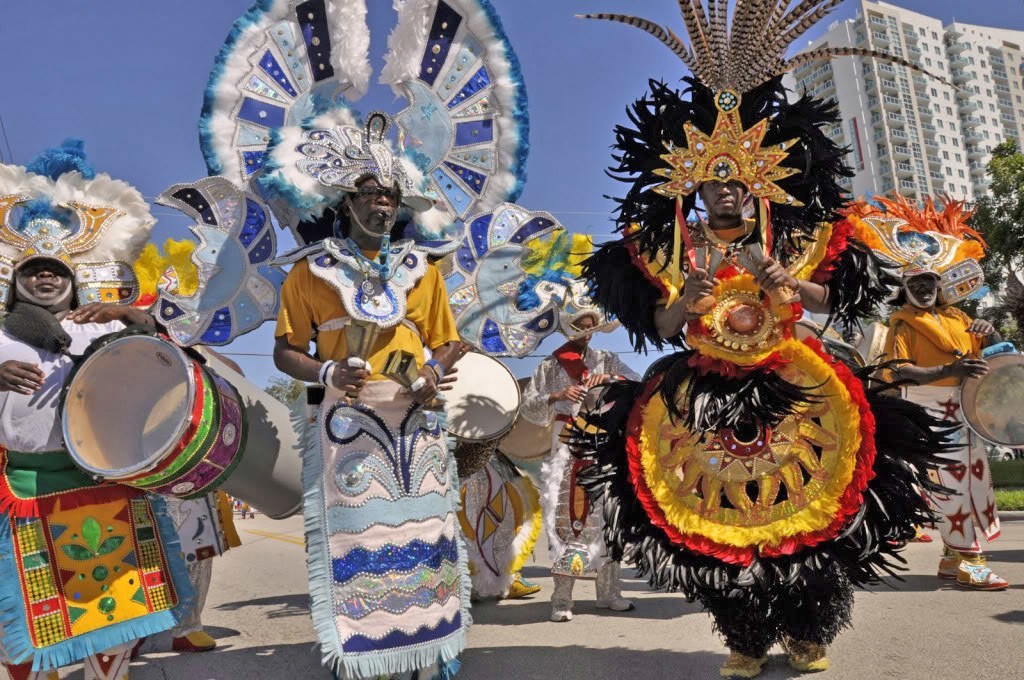In this vibrant outdoor parade scene, the sky is a clear blue with a large high-rise white building visible in the background, indicating a city setting. The participants, all with dark complexions, are standing on the street, adorned in elaborate, colorful costumes. One striking figure wears an ornate headdress that is white with blue accents, adorned with jeweled markings. He also sports a matching apron-style outfit in the same color scheme, and carries red, green, and purple instruments in front of him. Flanking him is another dancer clad in black feathers with peacock-like designs and a standout yellow and red bejeweled star on his headdress, culminating in a wide circular emblem with black feathers around his waist. The festive atmosphere is complemented by a trio in the background, playing large steel drums. The detailed and ornate costumes, combined with the celebratory energy, suggest this event is a grand parade or carnival, likely marking a significant cultural or holiday celebration.